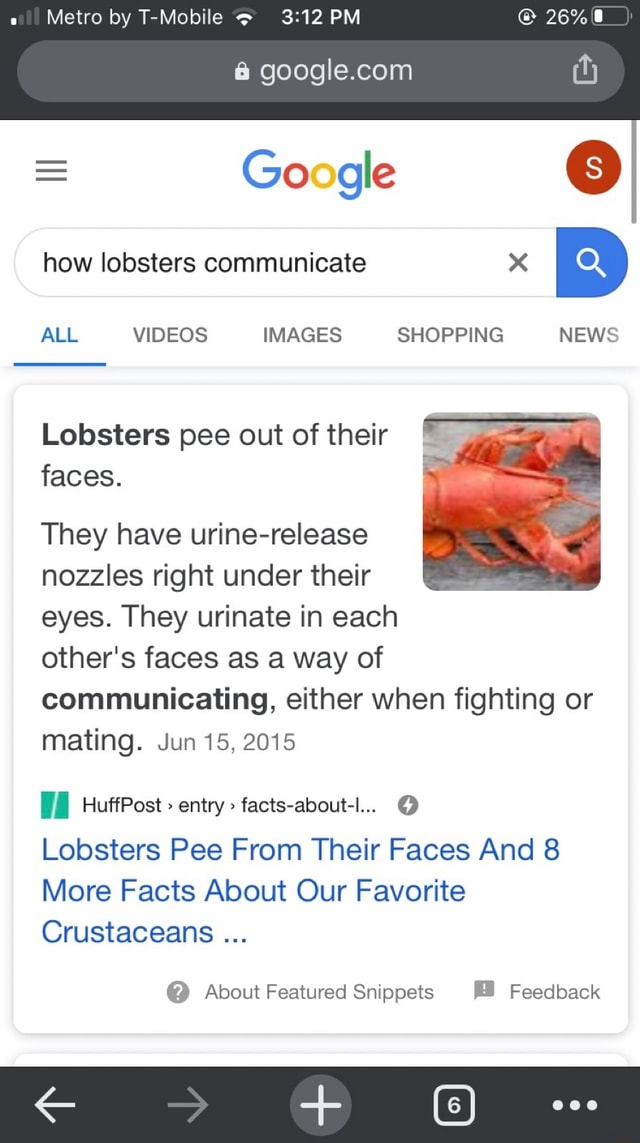The image depicts a Google search on a smartphone, indicated by the "Metro by T-Mobile" label at the top of the screen, alongside the time and battery life. The URL "google.com" is visible, and the Google logo is prominently displayed with the navigation menu icon (three horizontal bars) on the left. On the far right of the Google logo, a red dot accompanying an 'S' signifies the profile of the phone's user. The search query entered is "how lobsters communicate," within a search bar featuring a magnifying glass icon.

Below the search bar, various Google search categories are shown, including "All," "Videos," "Images," "Shopping," and "News." The top search result reveals an intriguing fact about lobsters: "Lobsters pee out of their faces." According to HuffPost, lobsters have urine release nozzles located just beneath their eyes and use this unique method of urination as a form of communication during fights or mating.

Additionally, the bottom of the phone's interface includes a navigation bar with an arrow, a plus mark, a box with the number six, and three vertical dots indicating additional options.